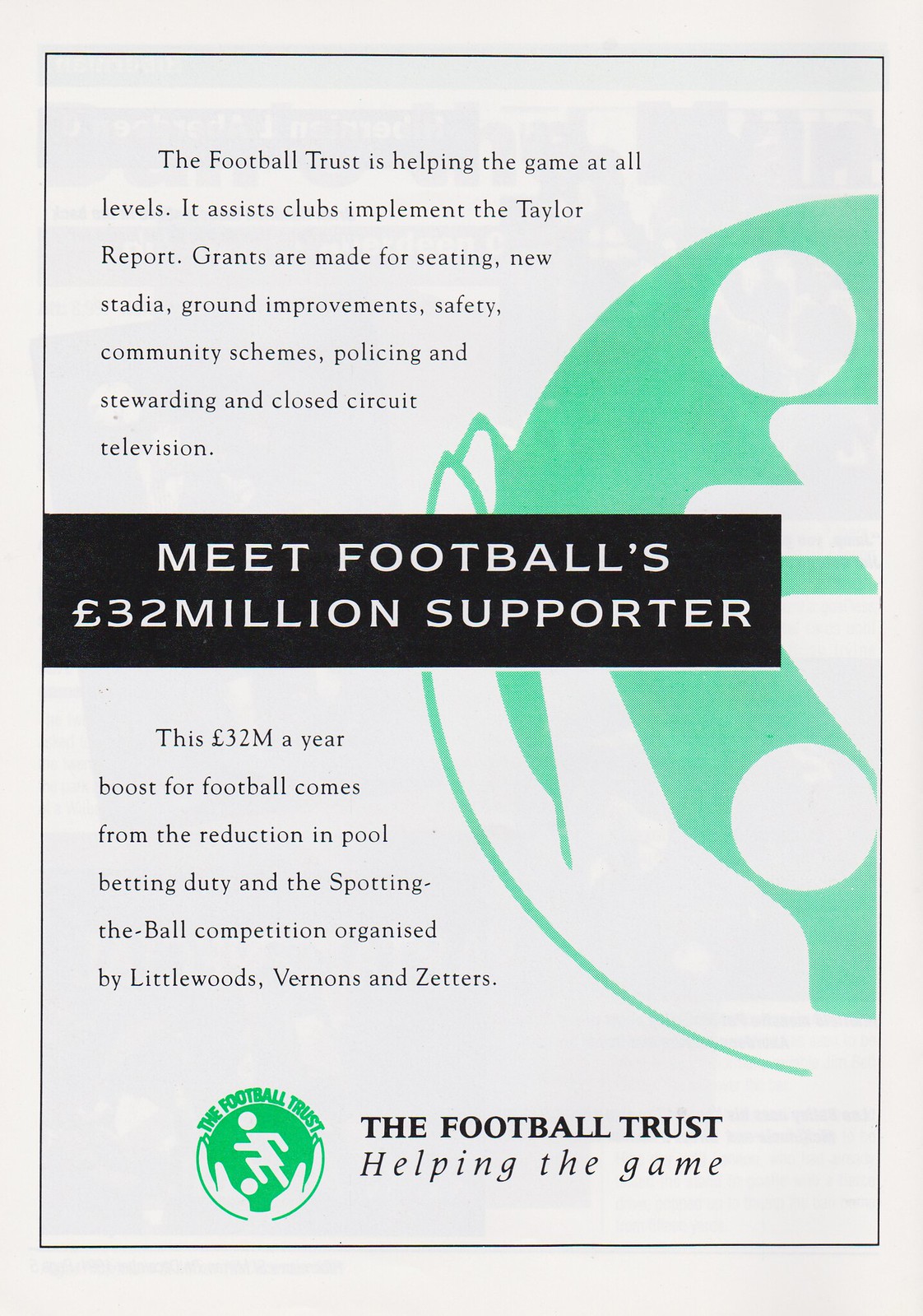The image is a detailed digital poster with a white background, prominently featuring a green logo on the right side, showing a light teal ball held by a white hand. The logo includes a white stick figure kicking a soccer ball, emphasizing the sport's essence. The poster's top third contains small black lettering stating, "The Football Trust is helping the game at all levels. It assists clubs in implementing Taylor Report grants." These grants support various initiatives such as seating, new stadiums, ground improvements, safety, community schemes, policing, and closed-circuit television (CCTV). Centrally, there's a large black rectangle with bold white text reading, "Meet football's £32 million supporter," highlighting the significant financial backing. The text follows a left-aligned orientation, continuing below, explaining that the £32 million annual boost for football is funded by a reduction in pool betting duty and a 'Spotting the Ball' competition organized by Littlewoods, Vernons, and Zetters. Finally, at the bottom, black lettering reiterates the commitment: "The Football Trust, helping the game."